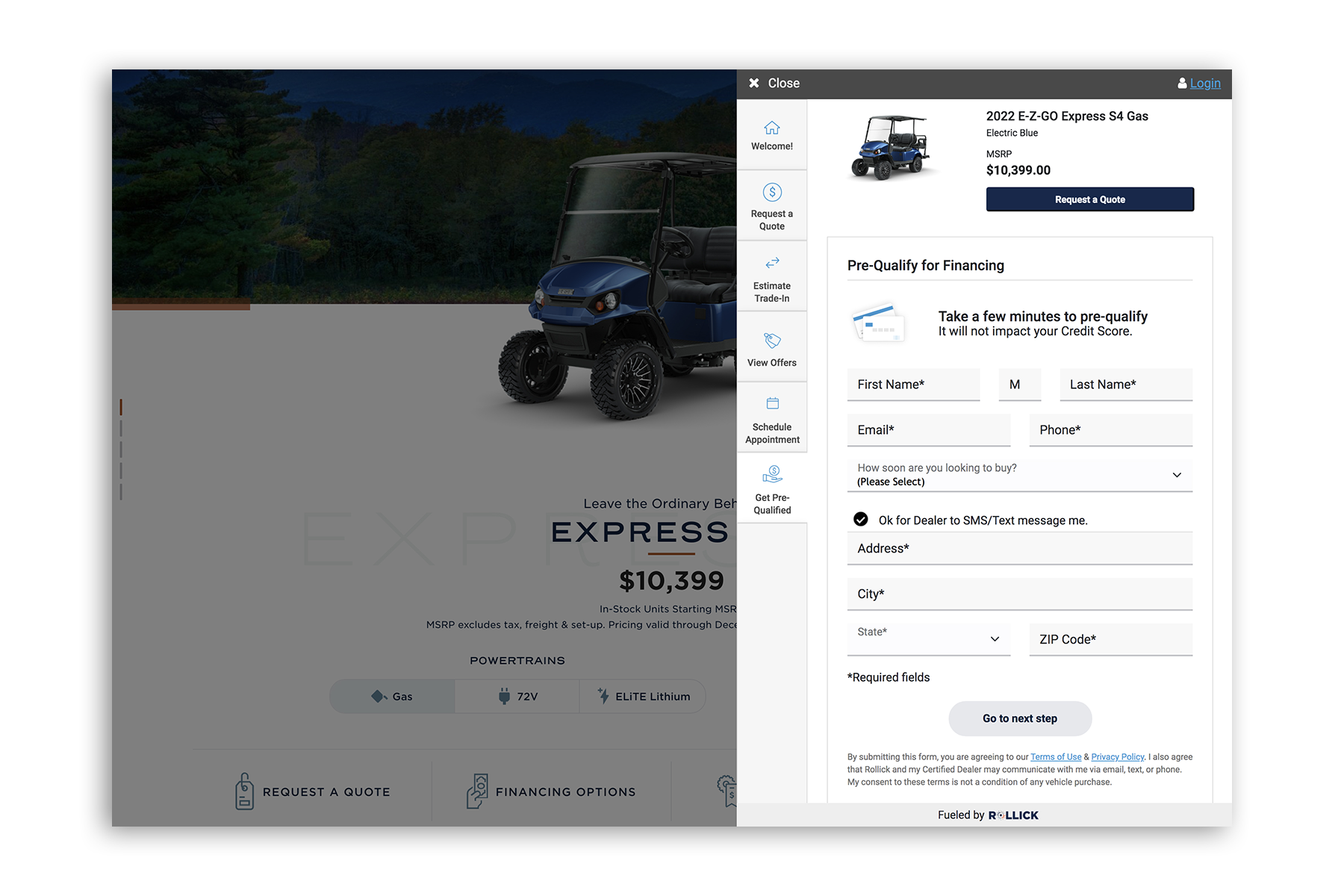A screenshot of a website dedicated to purchasing various types of small vehicles, particularly focusing on golf carts, is depicted. The primary focal point of the screenshot is a vibrant blue golf cart prominently displayed on the screen. This cart, identified as a 2022 EZGo Express S4 Gas, is highlighted as the product of interest and is listed at a price of $10,399.

In the background, a larger image of the same blue golf cart is visible, albeit slightly darkened to accentuate a pop-up sidebar that has appeared on the right side of the screen. This sidebar is lighter and more prominent to ensure visibility. At the top left of this sidebar, there's a close button, allowing the user to exit this view. Listed vertically within the sidebar are several actionable options: 

1. Welcome
2. Request a Quote
3. Estimate Trade-In Value
4. View Offers
5. Schedule Appointment
6. Get Pre-Qualified

Additionally, the screenshot provides a glimpse of the website's functionality and design: an inviting user interface meant to facilitate the purchasing and informational processes for potential buyers of golf carts.